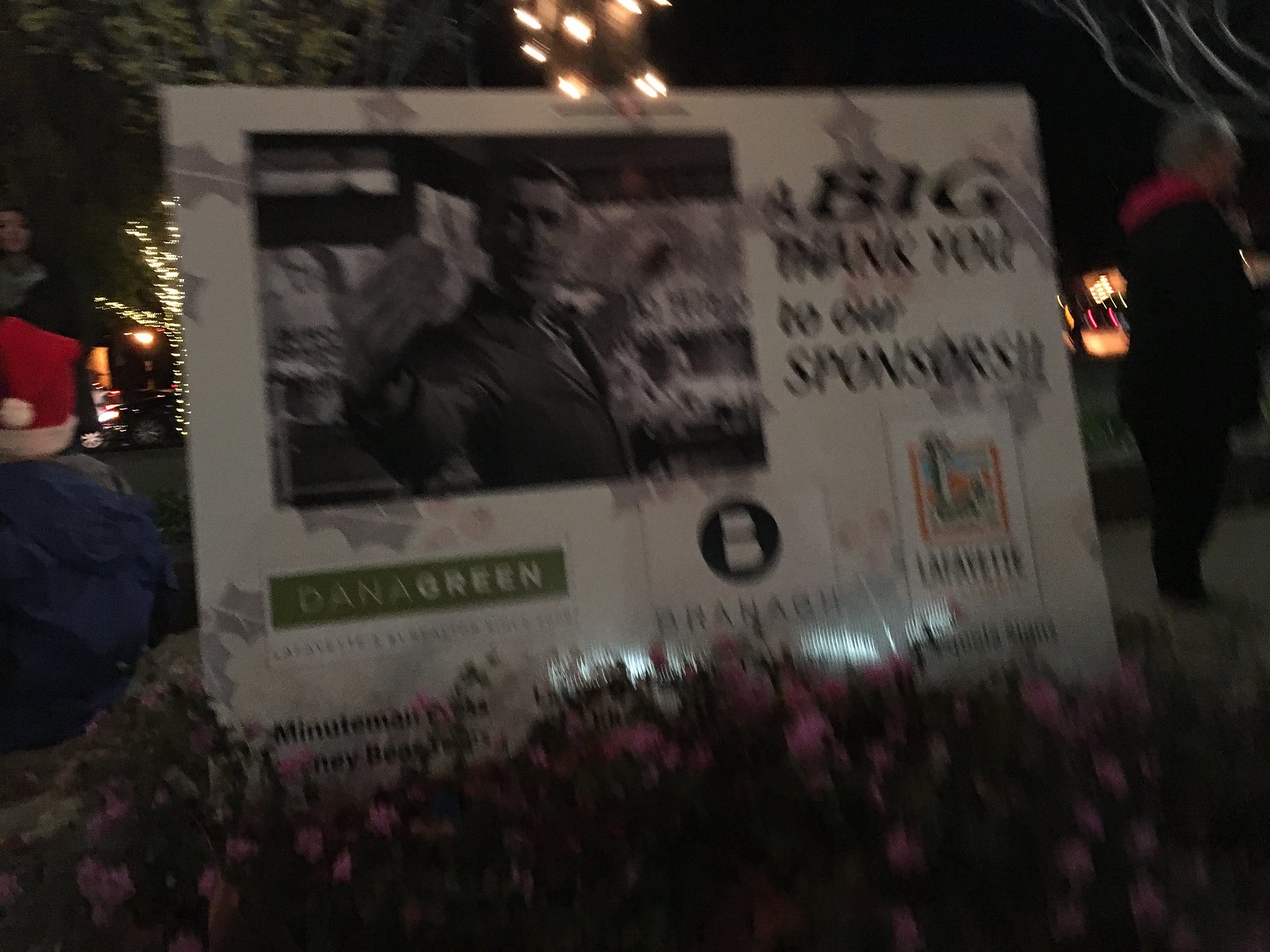In this photograph, an extremely grainy and blurry image captures a scene that appears to be set in a dark outdoor patio or dimly lit restaurant at night. The focal point is a large white poster board, tastefully surrounded by a bed of purple and white flowers at its base. Prominently displayed on the poster is an image of a man, likely a candidate or politician, depicted from the waist up. He is dressed in a suit with dark, slicked-back hair, and his arms are outstretched to his sides. To the right of his image, bold text reads: "A big thank you to our sponsor, Dana Green." In the background, the trees are adorned with twinkling lights, reminiscent of Christmas decorations, creating a cozy and festive atmosphere.